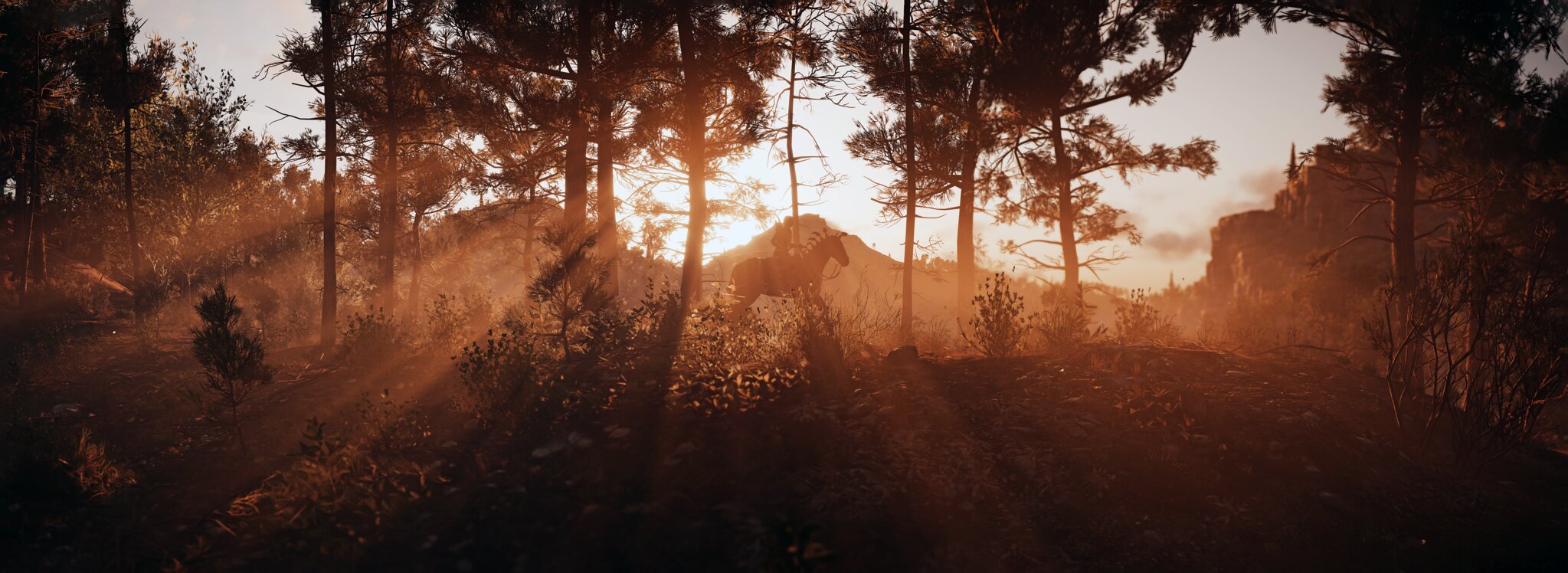The image, potentially a screenshot from a game such as Red Dead Redemption or an early morning landscape photograph, showcases a serene forested landscape bathed in a heavy sepia tint. Rays of sunlight, or god rays, shine through the pine trees on a gentle ridge, casting an orange glow and highlighting the scene with a reddish-brown hue. In the center, a person rides a horse from left to right, the horse's mane is distinctively spiky or braided. The rider and horse silhouette stand prominently among sporadically growing bushes and fully grown coniferous trees, positioned between two trees and illuminated by a sunray. The background features light grayish-lavender sky transitioning to mountain peaks and hilly areas in the distance, completing this picturesque morning scene devoid of other people or buildings.